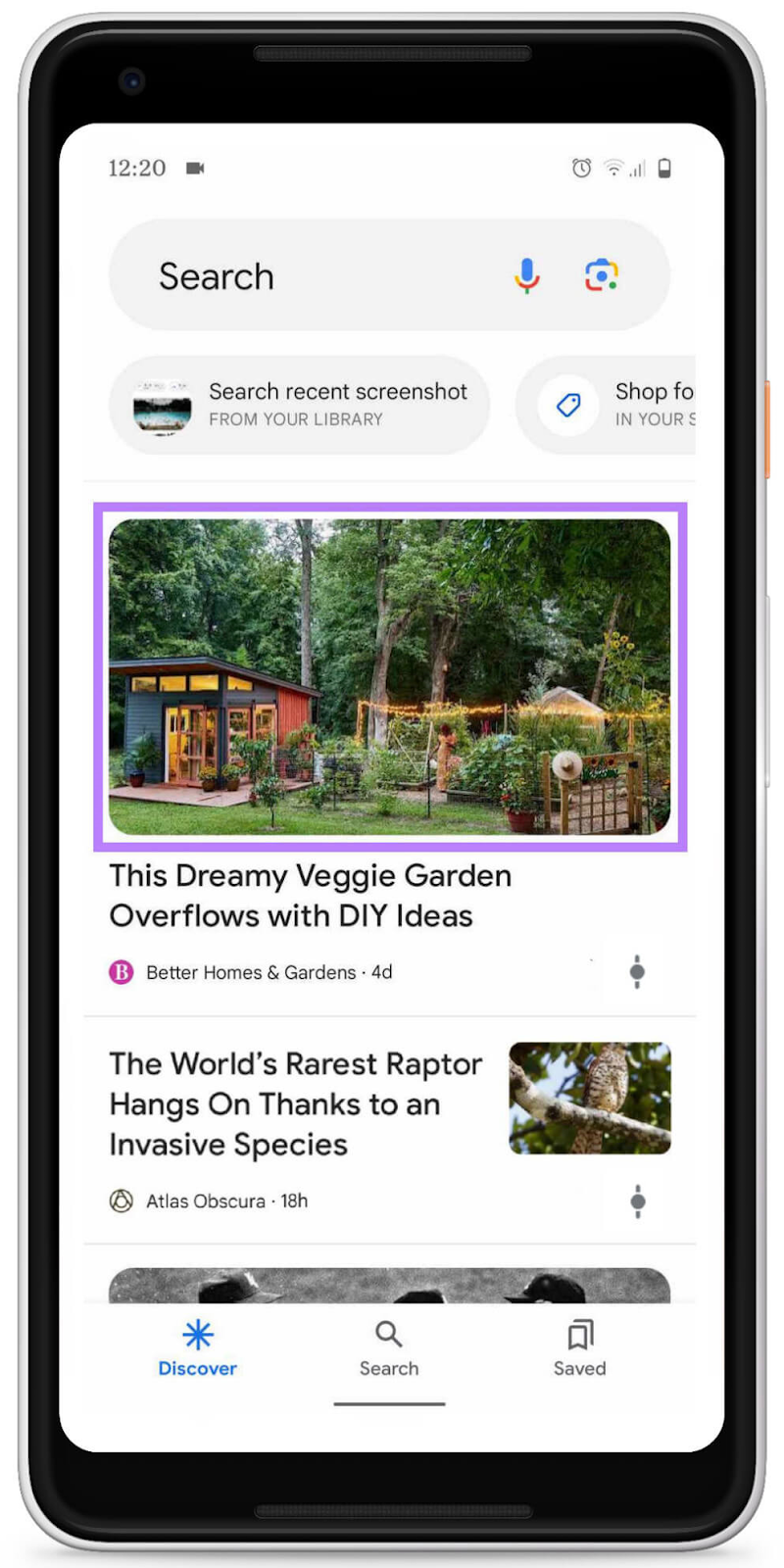This image is a detailed screenshot of a smartphone display on the Google app. At the top right corner, the battery icon is displayed vertically with approximately 20% remaining. To its left is the phone signal strength icon showing three out of four bars filled, followed by the Wi-Fi signal strength icon indicating only one out of four bars. Additionally, an alarm clock icon is present. 

On the top left, the time is clearly displayed as 12:20, with a dark gray video camera icon positioned to its right. Below this is a horizontal oval-shaped search bar area; the word "search" is written on the left in black, and on the right are microphone and camera icons. Beneath this, within a smaller oval, it reads "search recent screenshot from your library."

In the center of the image, there's a photo placed within a purple-bordered square. The photo depicts a forested area with numerous large green trees. A woman stands prominently in the lower part of the photo wearing a dress in shades of pink and yellow.